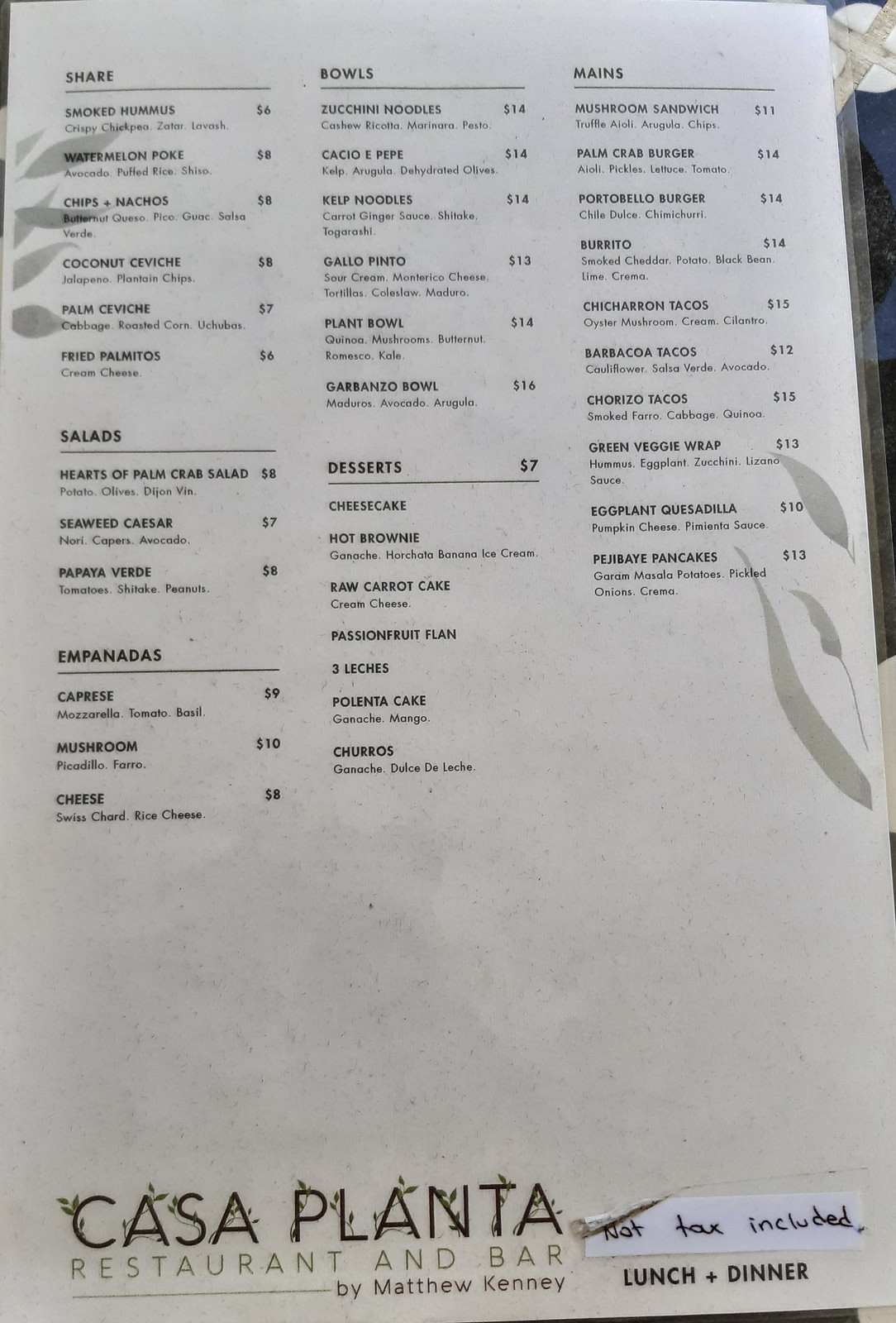The photograph showcases a detailed menu from "Casa Planta Restaurant and Bar by Matthew Kenney." The menu is elegantly presented on laminated white paper, adorned with subtle, stylized gray leaves and stems on the edges, imparting a natural aesthetic. The restaurant's name is prominently displayed at the bottom in an artistic font, with leaves artfully intertwined within the letters. Beneath the name, it specifies "Lunch and Dinner," with a small white paper note taped over it, indicating "Not Tax Included."

The menu is organized into several sections:

- **Appetizers Under "Share":** Smoked Hummus, Watermelon Poke, Chips and Nachos, Coconut Ceviche, Palm Ceviche, Fried Palmitos.
  
- **Salads:** Hearts of Palm Crab Salad, Seaweed Caesar, Papaya Verde.
  
- **Empanadas:** Caprese, Mushroom and Cheese.
  
- **Bowls:** Zucchini Noodles, Cacio e Pepe, Kelp Noodles, Gallo Pinto, Plant Bowl, Garbanzo Bowl.
  
- **Desserts:** Cheesecake, Hot Brownie, Raw Carrot Cake, Passionflower Flan, Tres Leches, Polenta Cake, Churros.
  
- **Main Entrées:** Mushroom Sandwich, Palm Crab Burger, Portobello Burger, Burrito, Chicharron Tacos, Barbacoa Tacos, Chorizo Tacos, Green Veggie Wrap, Eggplant Quesadilla, Paje Pancakes.

The menu's overall design and layout not only emphasize the restaurant's commitment to creativity and detail but also hints at a culinary focus on fresh, plant-based ingredients curated by Matthew Kenney.